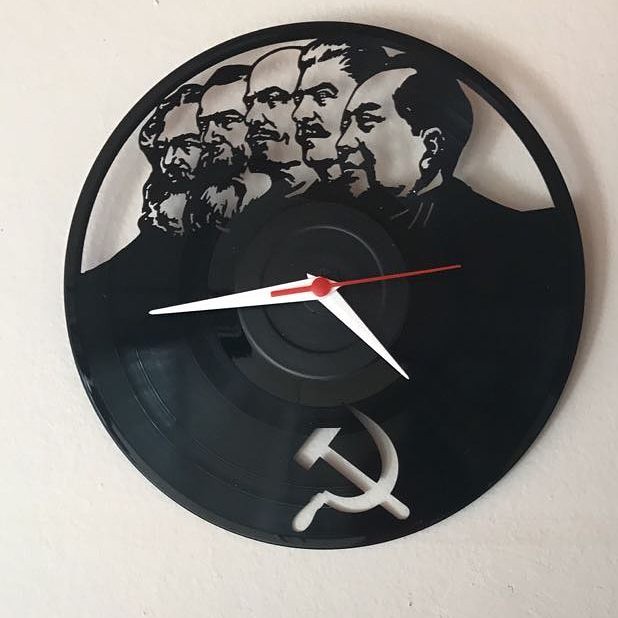This unique wall clock features a black vinyl design that ingeniously mimics the appearance of a vinyl record. At its center, a bold white hammer and sickle symbol stands out prominently. The clock’s minimalist face is devoid of numbers, highlighting its modern and unconventional aesthetic. Time is marked by three sleek hands: a thin red second hand, a short white hour hand, and a longer white minute hand. Intricately carved along the top edge are figures of five influential individuals known for their communist ideologies. From right to left, identifiable faces include Mao Zedong and Joseph Stalin, with three other prominent yet unnamed individuals completing the ensemble.